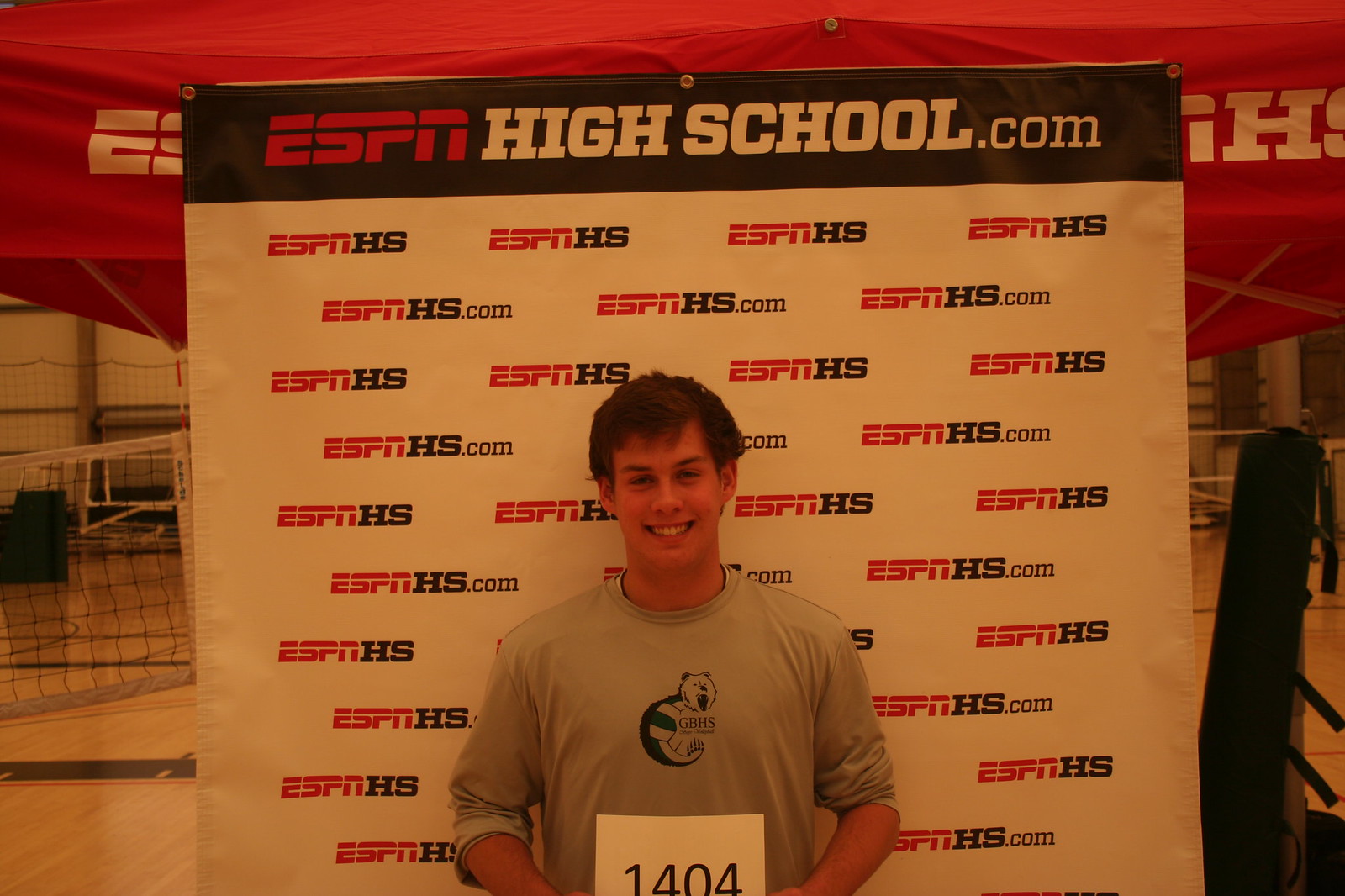This horizontally framed photograph captures a smiling young man standing waist up in a gymnasium. The gym has a distinctive light brown wooden floor and a volleyball net visible on the left side. In the center, the young man, a white teenager with short, roughed-up brown hair, is posing confidently. He's dressed in a long-sleeve gray shirt with the sleeves rolled up to his elbows, emblazoned with the logo of a bear and the acronym "GBHS." Behind him, an eye-catching white banner stretches across the background, featuring a black bar at the top with the red text "ESPNHIGHSCHOOL.COM" and a repeating pattern of "ESPNHS" and "ESPNHS.COM" in rows. Just behind him, there's also a red canopy tent that partially shows the ESPN logo. In his hands, he holds a white piece of paper with the number "1404" printed in black. This detailed composition highlights both the individual and the vibrant sports culture around him.